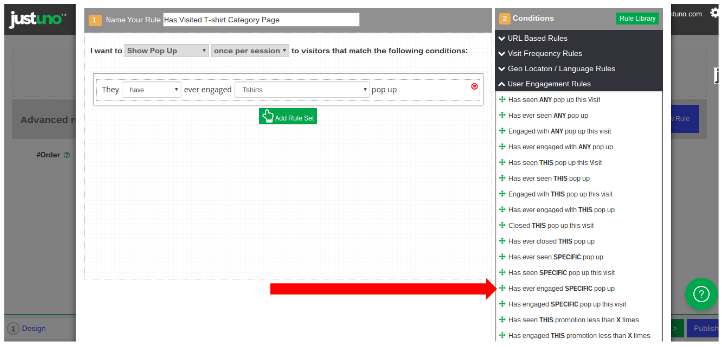In the detailed image description, the left corner features the word "JUST" in white text merged with "UNO" in green text, forming a single combined logo. Moving slightly to the right, there's a search bar with placeholder text indicating "Name of the rule." This search bar is on a page showing the "t-shirt category." Below this, a gray rectangle presents options labeled "I want to show pickup" once per session to visitors who meet specific conditions.

To the left, a new, finely outlined rectangle is evident. It's segmented with tiny lines and contains the word "They" accompanied by a downward-pointing arrow. Inside another similar rectangle, there's a downward arrow with the term "engaged" next to it, and yet another with "t-shirts."

Adjacent to these elements, there is a green rectangle with the word "pop-up." Beneath this, another green rectangle reads "Add rule set," indicated by an upward-pointing finger icon.

On the right side of the image, "conditions" is prominently displayed. Additionally, a green rectangle within this area features the text "Mute library." Below this, there are selections against a black background, including "URL based," "Visit frequency rules," "Geolocation-language rules," and "User engagement rules."